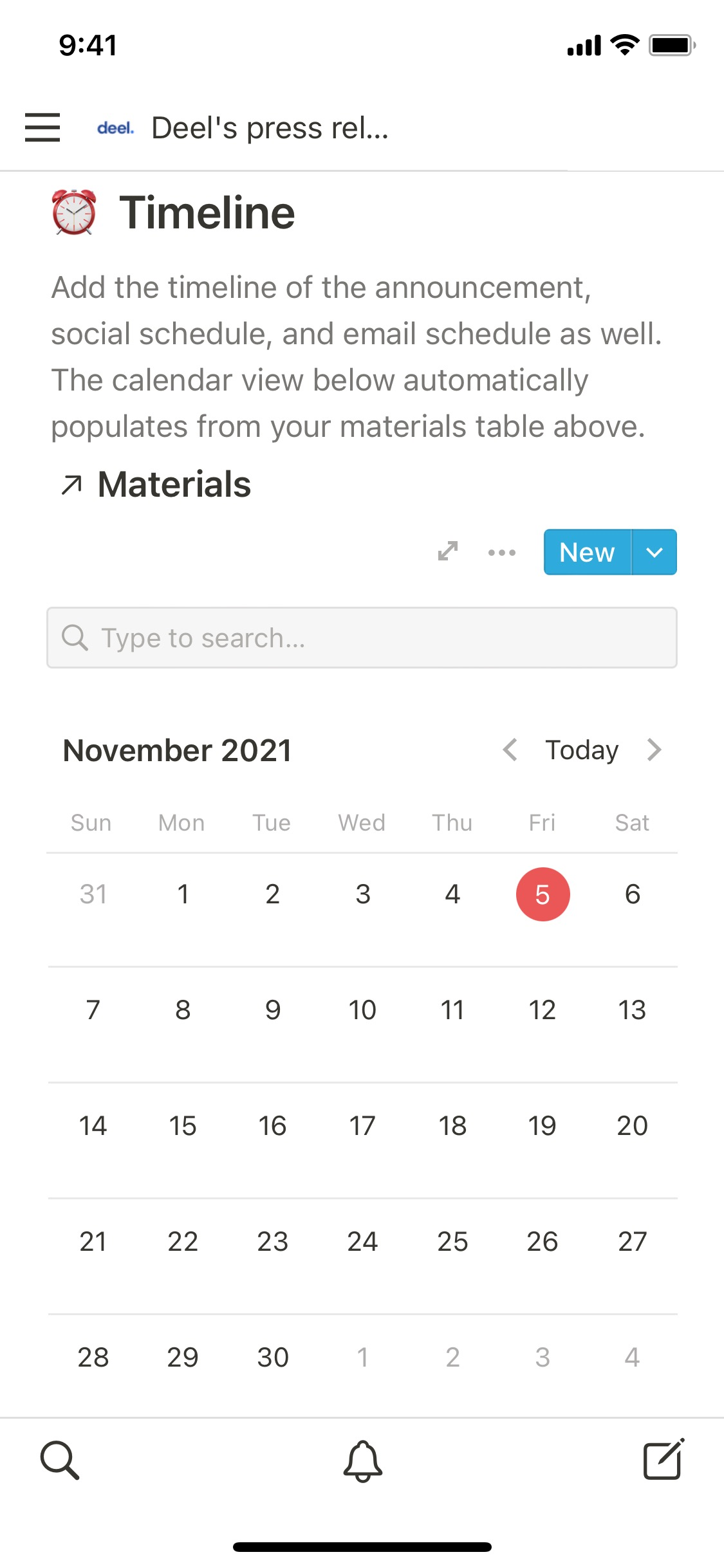**Detailed Caption:**

The screenshot showcases a mobile application interface titled "Deal," captured at 9:41 (unclear if it's a.m. or p.m.). The status indicators display a full network signal and a fully charged battery at the upper right corner.

At the top of the interface, the application is focused on a section labeled "Deals Press REL...", presumably short for "Press Release Calendar." The header "Timeline," adorned with a red clock icon, indicates the main feature of the screen.

The descriptive text in the top section reads: "Add the timeline of the announcement, social schedule, and email schedule as well. The calendar view below automatically populates from your materials above," which is clarified by an upward-pointing arrow linked to another header labeled "Materials."

Further down, there are buttons for expanding the view, viewing options, and creating new items, with a drop-down menu available. Below these options is a search bar with the placeholder text "Type to search." The calendar display for November 2021 is prominently featured, with a red circle highlighting Friday the 5th, marking it as "Today."

In the bottom navigation bar, there are several icons: a magnifying glass for search on the left, a bell icon in the center likely used for setting or reading notifications, and an icon on the lower-right corner for creating or writing new entries. This implies adding new items to the press release calendar, aiding in the scheduling of content.